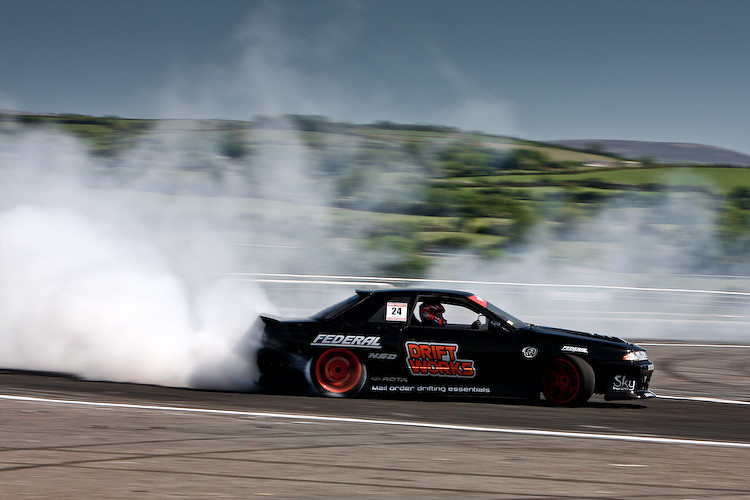The photograph captures a high-speed black racing car skidding on a gray asphalt road, emitting a cloud of white smoke from its burning tires. The car, which features contrasting red rear wheels and black front wheels, displays the word "FEDERAL" underlined in white on the back right side and "DRIFT" in red. A piece of paper with the number "24" is visible in one of the rear windows. A driver, identifiable by a red and gray racing helmet, is maneuvering the vehicle. Above the scene, the sky is a deep blue, suggesting daylight. The background consists of rolling hills adorned with fields of grass, trees, and sparse vegetation, reminiscent of farmlands or pastures, presenting a serene countryside landscape. The road is marked with solid white lines along its edges, indicating a designated racetrack.